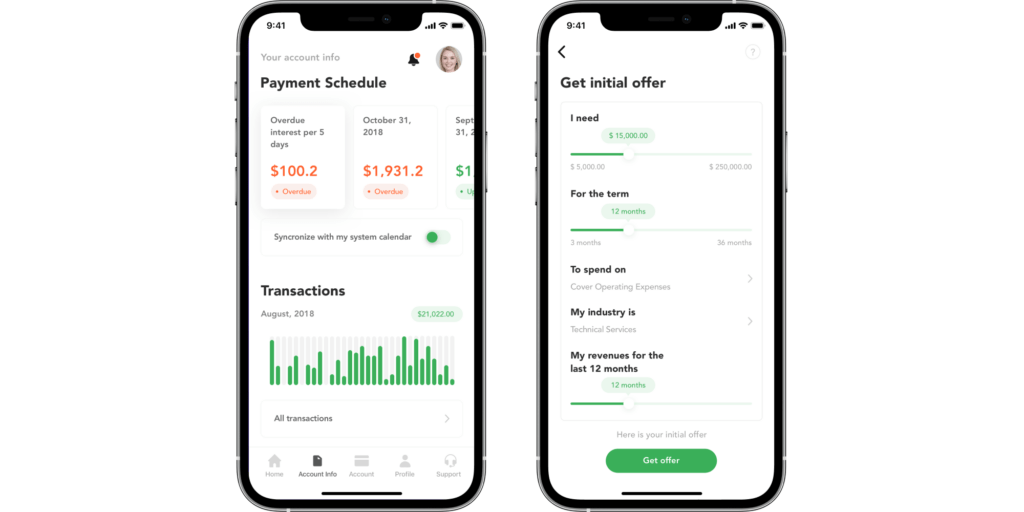### Detailed Caption for Image of Two Mobile Phones

The image showcases two mobile phones side by side, each displaying different screens of what appears to be the same financial app.

#### Left Phone Screen:
- **Payment Schedule Section:** 
  - Three boxes listing different payment details.
    - **Box 1:**  
      - **Overdue Interest:**  
        - **Details:** $100.20 overdue for 5 days  
        - **Visual Indicator:** Orange highlight
    - **Box 2:**  
      - **October 31st, 2018:**  
        - **Details:** $1,931.20 overdue  
        - **Visual Indicator:** Orange highlight with an "Overdue" tag below
- **Synchronize with My System Calendar:** This option is toggled on.
- **Top-Right Corner:** Features an avatar of a woman and a bell icon.
- **Transactions Section:**
  - A bar chart depicting transactions data starting from August 2018.
  - **Highlighted Transaction:**
    - **Tag:** $21,022 on the right side
    - **Footer:** Label that says "All Transactions"

#### Right Phone Screen:
- **Get Initial Offer:**
  - **Interactive Chart:**
    - **Adjustable Green Line:** Allows the user to increase or decrease the values.
  - **Loan Options:**
    - **Amount Needed:** Ranges from $5,000 to $250,000, currently set at $15,000.
    - **Term Duration:** Spanning from 3 months to 36 months, currently set at 12 months.
  - **Additional Information:**
    - **Usage:** To cover operating expenses.
    - **Industry:** Technical services.
    - **Revenue:** Configured for the past 12 months.
  - **Button at Bottom:** Green button labeled "Get Offer".

Together, these two screens provide comprehensive functionalities of a financial management app, including monitoring overdue payments and generating loan offers based on user preferences.